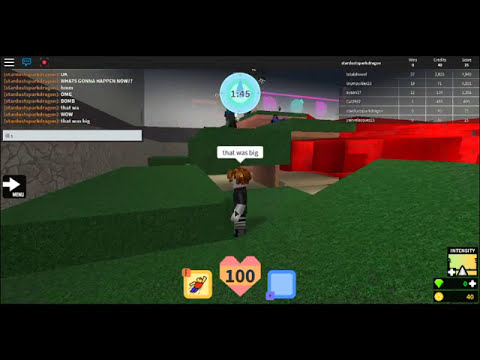In the image, we see a screenshot from a video game with a blocky, Minecraft-esque aesthetic. The central character, who has brown shaggy hair and grayish skin, wears a blue shirt and dark blue pants. He stands on a slanted, green grassy area with blocky walls and a red building in the background. Above his head, a white text box reads "That was big," and there's a blue timer that shows 145 in black numbers. Just below him, a pink and yellow heart, displaying 100, represents his health. To the left, there's a yellow icon of a person in a flying pose with a "1" next to it, indicating a superpower. On the right, a blue box appears empty. In the top-right corner, there's a black-and-white scoreboard, while the bottom-left features a purple circle, a green diamond with a zero counter and a plus sign, a gold coin symbol showing 40 coins, and a green-to-gold level counter. Despite the clutter, the scene is set on layered, green grass with gray stone walls and a red floor area in the background.